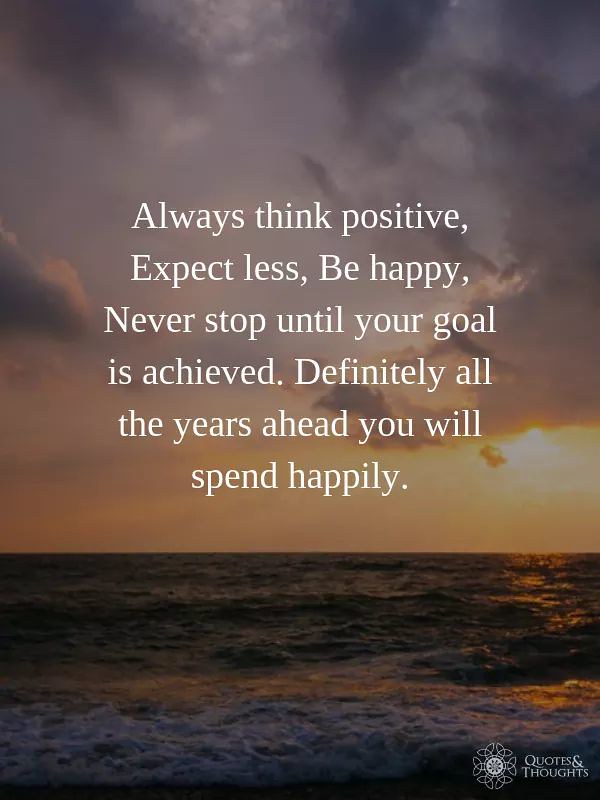The image resembles an inspirational poster with a vertical rectangular shape featuring an ocean setting. The sky is partly cloudy, displaying a mix of hazy and wispy puffy clouds. The sun is either rising or setting, casting a fiery yellow glow on the horizon that transitions into pink and then a darker grayish-blue at the top. The ocean occupies the bottom third of the image with gentle waves reaching the beach. In the lower right corner, a white logo with a flowery mandala design is accompanied by the words "quotes and thoughts." The main quote, centered in white text, reads: "Always think positive. Expect less. Be happy. Never stop until your goal is achieved. Definitely, all the years ahead, you will spend happily."